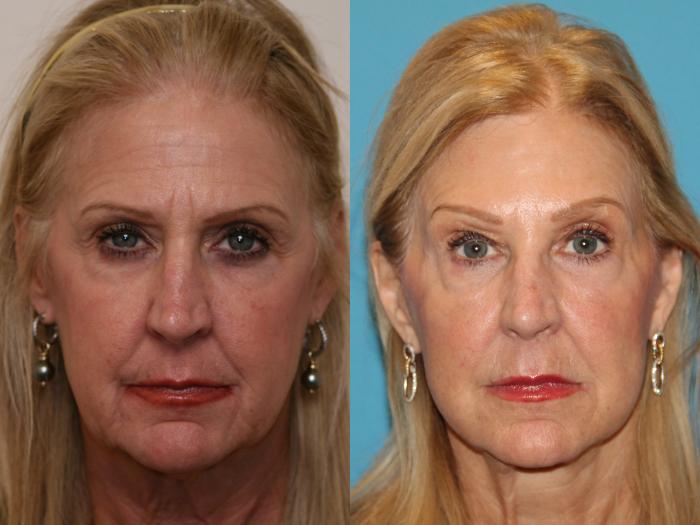This image features side-by-side close-up photos of the same woman, possibly in her 50s or 60s, with dyed blonde hair and fair skin. In both photos, she is wearing eye makeup and reddish lipstick, and she has blue eyes. She is also adorned with dangling silver and gold earrings in each shot, although they appear slightly different. 

In the left photo, she wears a yellow headband, and the lighting is darker, casting a shadow over her face, which emphasizes wrinkles and gives her an older appearance. The background in this photo is gray. On the right, the lighting is much brighter, making her face appear smoother and younger with fewer visible wrinkles. The background here is blue. Despite the differences in lighting and backdrop, her expression remains neutral in both photos, and she gazes directly into the camera. The contrasting lighting and settings suggest that these images might be depicting a before-and-after scenario, possibly related to cosmetic changes or plastic surgery.